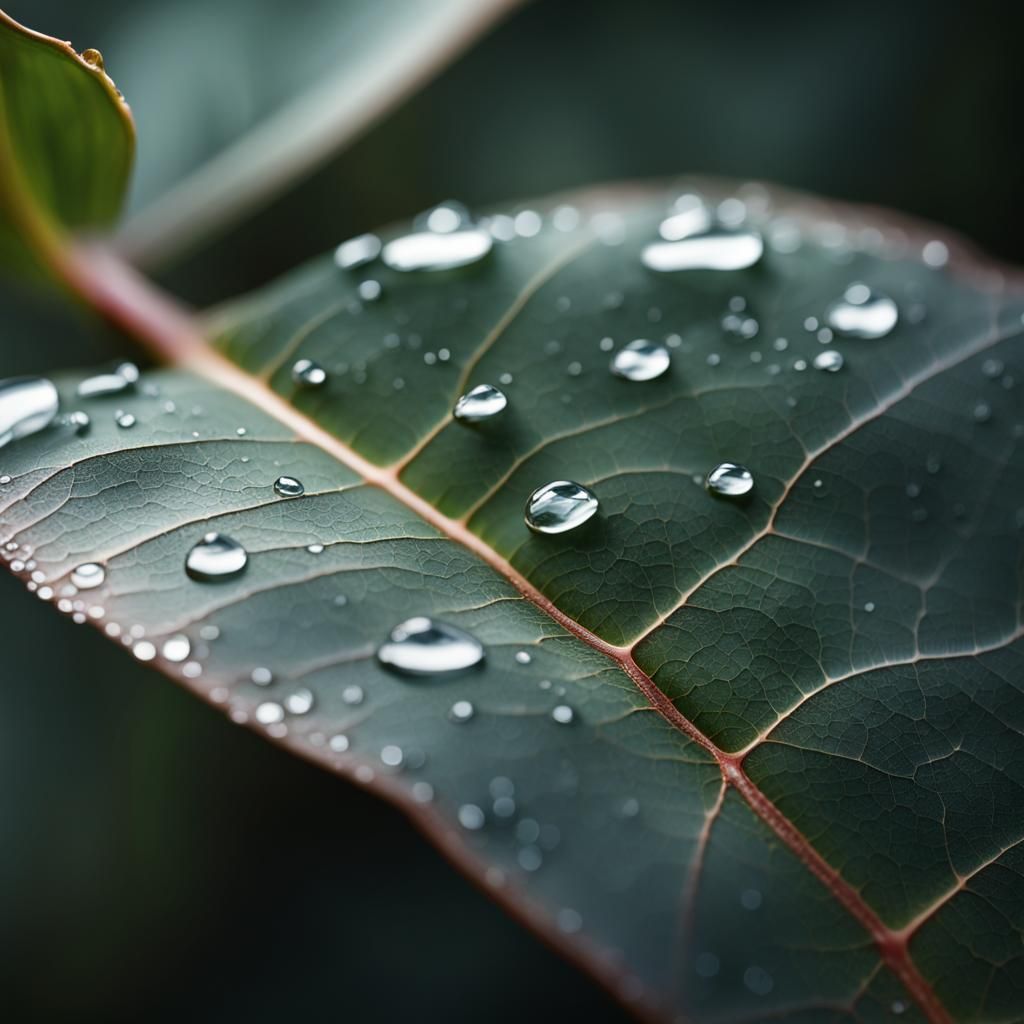The image is a close-up, high-resolution photograph of a single dark green leaf, slightly taller than it is wide. The leaf is covered in numerous, crystal-clear water droplets of various sizes, with smaller droplets clustering around the edges. The central vein of the leaf, which creates a prominent "alleyway" down the middle, is visible with some cracks and branching veins that are a brownish-reddish color. The leaf appears thick and textured, with these veins providing a stark contrast to the green surface. The background is out of focus and transitions from a dark, almost black hue at the bottom left to a lighter green towards the top and right, giving it an abstract feel. This blurring effect emphasizes the leaf's detailed structure and the pristine clarity of the water droplets.